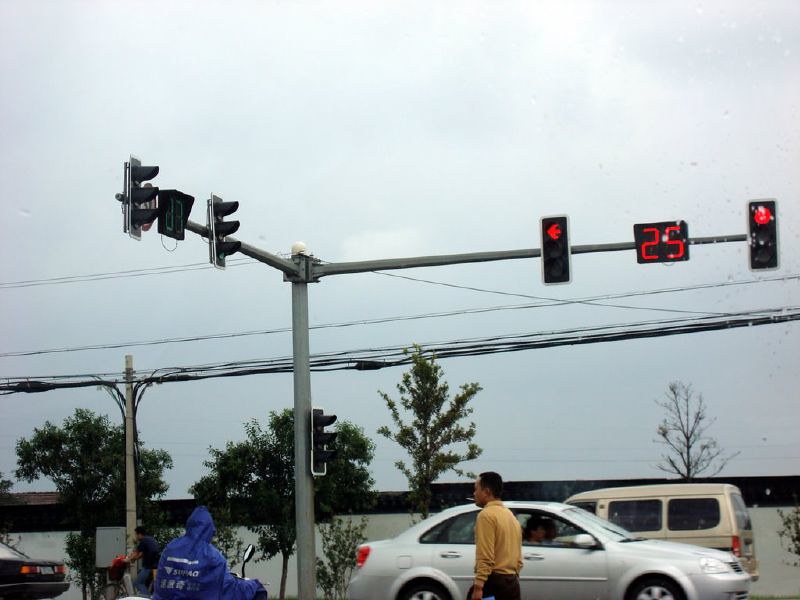The photograph was taken outdoors on a cloudy, rainy day and features a notable traffic light system. Prominently, there is a traffic light with four lights in total. The top light is a red arrow pointing left, and below it is a red light with the number "25," likely indicating a speed limit. Further down are two more traditional circular signal lights, also currently red. The traffic lights are mounted on a metal pole with a long arm extending to the right, equipped with light hoods to prevent misreading.

In the background, a white building with a black border on top can be seen, accompanied by several trees—some with leaves, but a couple without. Additionally, there are power poles with numerous black wires strung tightly between them.

On the highway in the foreground, three cars are visible: a silver car pointed to the right, a gold minivan to the left, and the back of a black car heading left. A person wearing a blue raincoat is sitting down, likely on a motorcycle or moped, while another person dressed in a long-sleeved tan shirt and black pants is walking toward the seated individual. The scene notably lacks any text or words, providing a clear snapshot of a typical rainy day at a traffic intersection.